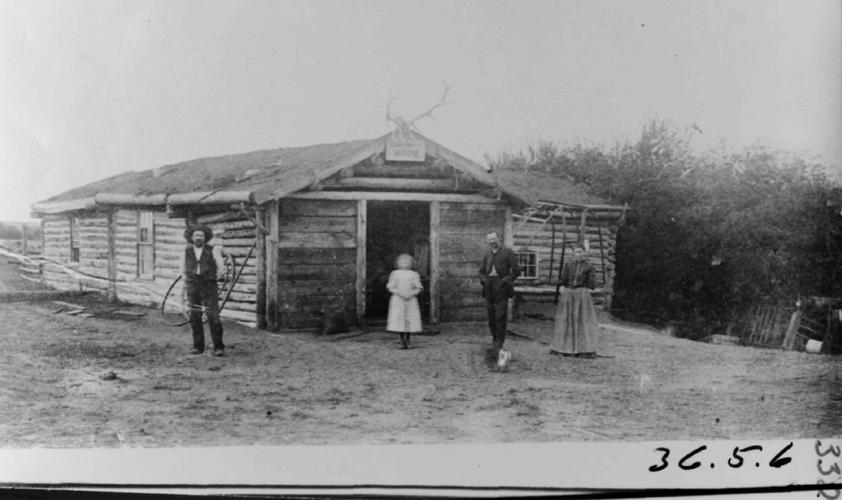This is a very old black-and-white photograph, reminiscent of the late 1800s or early 1900s, capturing a rundown shack on a barren farm, likely in the Old West of the US. The image features four figures standing outside the wooden house: two men, a little girl, and a woman. To the left stands a bearded man dressed in black pants, a white shirt, a black vest, and a hat. Centered in the doorway is a little girl in a white dress. Adjacent to her on the right is another man wearing black pants and a dark jacket with his hands in his pockets. To the far right is a woman in a long, flowy skirt and a long jacket. The background shows sparse shrubbery and bare dirt with no grass. Dominating the top of the cabin's roof are two large antlers. The bottom right corner of the photo is marked with the numbers 365.6 and 332 handwritten, and there's an illegible sign attached to the cabin.